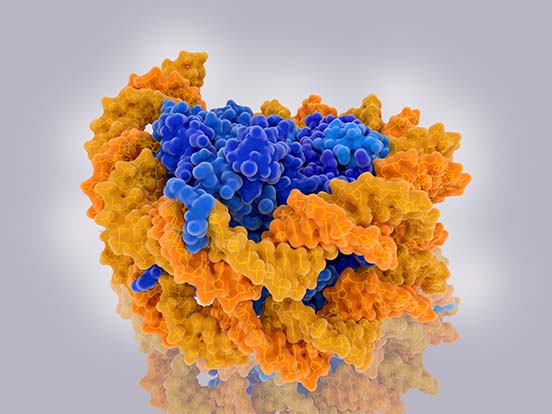This image presents a vibrant, intricately detailed structure set against a gray background with slight light filtering through. The photograph appears to capture a complex object, potentially resembling a microscopic scene of bacterial colonies or a biological model. Central to the object, there is a russet or gold, spiky surface interwoven with orange and orange-yellow elements, suggesting a colony or clusters intertwined with each other. The center features clusters of blue, bead-like shapes, predominantly gathered at the top but dispersed throughout the object. The reflective surface beneath creates a mirrored effect, enhancing the image's depth and contrast. The vivid yet somewhat muddy colors of orange, gold, and blue stand out sharply against the gray backdrop, suggesting a blend of artistic representation and scientific visualization.